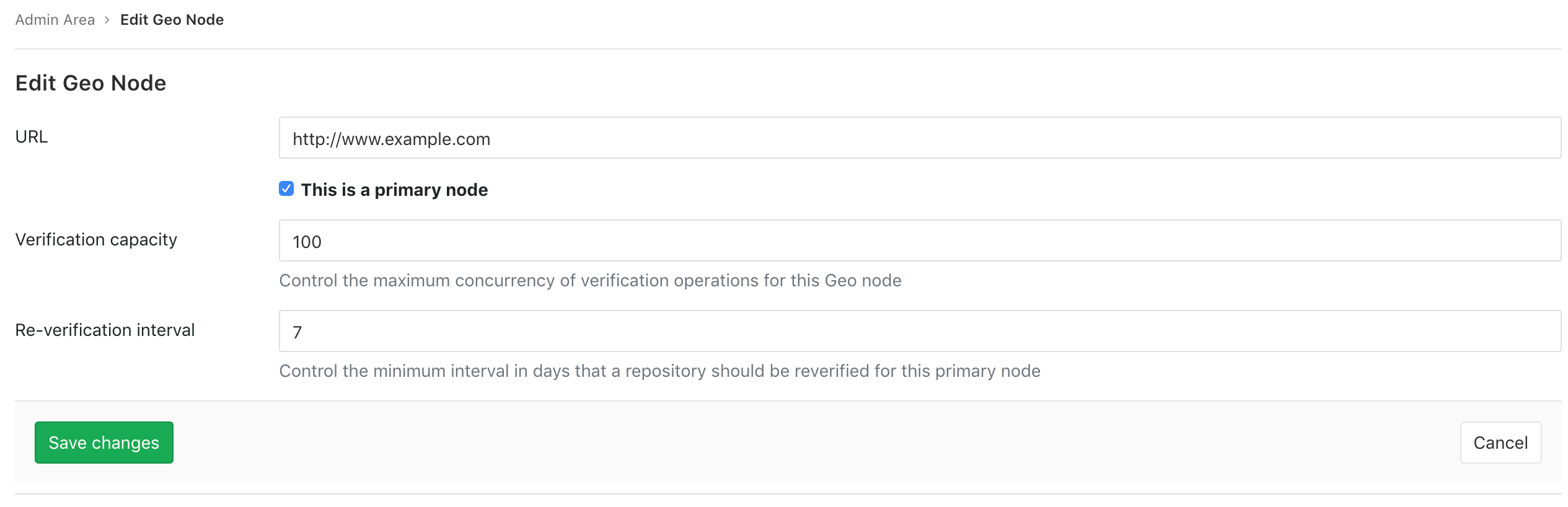**Detailed Description of the "Edit Geo Node" Section in the Admin Area of a Website:**

This image captures a screenshot of the "Edit Geo Node" section located within the admin area of a website. The screenshot does not reveal the name or the specific details of the website, focusing solely on the administrative editing interface. The entire background is stark white, providing a clean and minimalistic visual appeal.

At the bottom of the page, there are two distinctive buttons placed at opposite corners. On the left-hand side, a prominent green button labeled "Save Changes" stands out, indicating its functionality with clear intent. Conversely, on the right-hand side, a white button labeled "Cancel" provides an option to abort any changes made.

Within the "Edit Geo Node" section, there are three primary editable options:
1. **URL**: The first editable field designated for the URL currently contains a placeholder text: "http://www.example.com." This placeholder suggests that no specific URL has been entered yet.
2. **Primary Node**: Adjacent to the URL field, there is a checkbox option labeled "This is a primary node," which can be either checked or unchecked based on the administrative decision.
3. **Verification Capacity**: The next editable field specifies the "Verification Capacity," which is set to 100. Below this field, an explanatory note clarifies that this setting controls the maximum concurrency of verification operations for this geo node.
4. **Re-Verification Interval**: The final option available is the "Re-Verification Interval," set at seven days. The accompanying description indicates that this setting manages the minimum interval in days required for the repository to be re-verified for the primary node.

Overall, the interface is simplified for ease of use, aimed at facilitating efficient administrative control of geo nodes within the website's backend system.